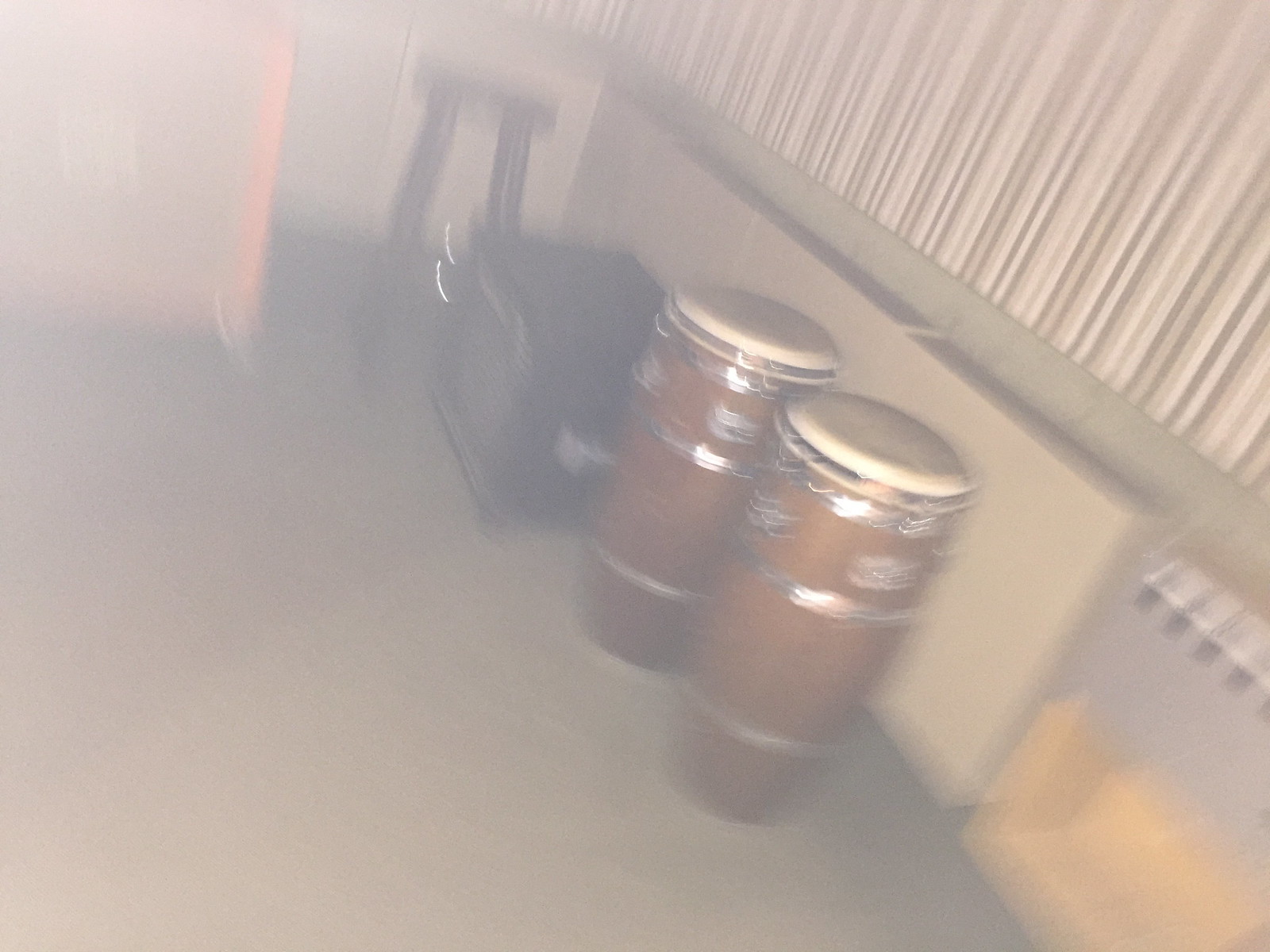A grainy, low-resolution photo captures the interior of a modest room. In the foreground, two well-worn bongos with natural wooden frames and white drumheads stand on a flat, gray floor. The drumheads show signs of extensive use, covered with smudges and marks where hands have rhythmically beaten them. Metal brackets encircle the wooden frames, adding structural integrity and visual interest.

The bongos rest against a plain white wall, which features a decorative border running along its midpoint. Above this border, the wall boasts a striped pattern that encircles the entire room, adding a touch of design to the otherwise simple space. 

To the rear of the bongos, a black amplifier with a white front panel sits quietly, hinting at a musical environment. Further along the same wall, a stool can be seen, suggesting a space used for musical practice or casual seating. The entire image is obscured by a white haze, adding a sense of nostalgia and making it difficult to discern fine details.